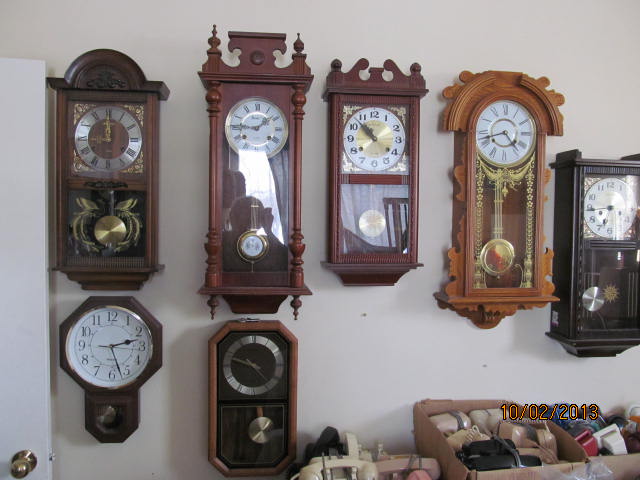This is a color photograph depicting seven antique wall clocks, meticulously arranged against a light grey wall with the shadows indicating a light source from the right. The majority of the clocks are framed with dark wood and display intricate designs, particularly at their tops. The clocks are arranged in two rows; the top row consists of five rectangular clocks while the bottom row houses two uniquely shaped ones: an octagonal clock with a smaller section below and an elongated hexagonal clock featuring an aluminum-outlined circular face. Each clock has a pendulum in various shades of gold, silver, and white.

The majority of the clock faces are white, with the exception of a silver and brown faced clock on the left. Notably, the clocks display different times. The background shows a partial view of a white door with a gold doorknob at the bottom left corner. At the bottom right corner, there is a cardboard box containing various small items in black, cream, blue, and red, which appear to be fabrics or small plastic items. Beside this box, there are two smaller piles of items in cream and pink. Additionally, old corded telephones in boxes are visible beneath the clocks. A date stamp, either October 2nd or February 10th, 2013, is present, marking the moment captured in the photograph.